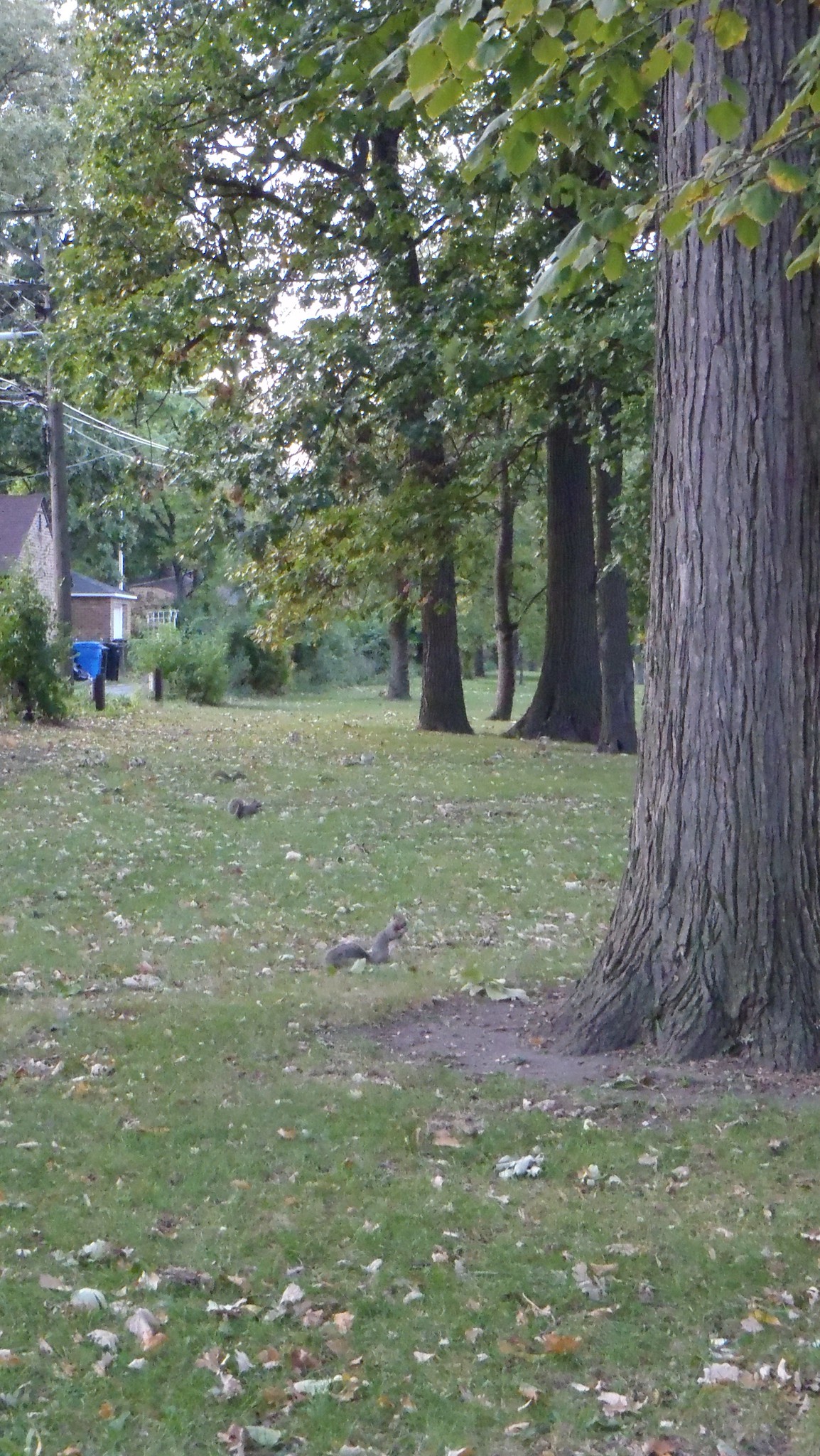The photograph captures an outdoor scene in what appears to be an expansive green field with tall, stately trees that seem to be maples, given their wide, green leaves. These trees dominate the scene, spreading their branches and foliage that drape down, creating a dense canopy. The trunks of the trees are a gray-brown, blending seamlessly with the brown squirrels scattered across the ground. These squirrels, three in number, are foraging for food amongst the grass and dried leaves, indicative of early autumn. The scene contrasts with the vibrant green of the grass and trees against the brown and orange hues of the fallen leaves and tree trunks.

In the background, several small houses can be seen without back fences, suggesting they open up into this green belt area. The homes are primarily constructed from red brick and are flanked by green bushes and adorned with blue and black garbage bins. Additional elements include a brown wooden power line pole with electric wires and a bright, cloudy sky that casts a white light over the panorama. This scene is further detailed with sporadic patches of dirt amongst the grass and a porch visible to the left side, near which a small, mysterious blue box and additional bushes can be observed. This serene, natural setting, teeming with wildlife, is framed by a mix of residential elements and autumnal touches, creating a picturesque blend of nature and suburban life.